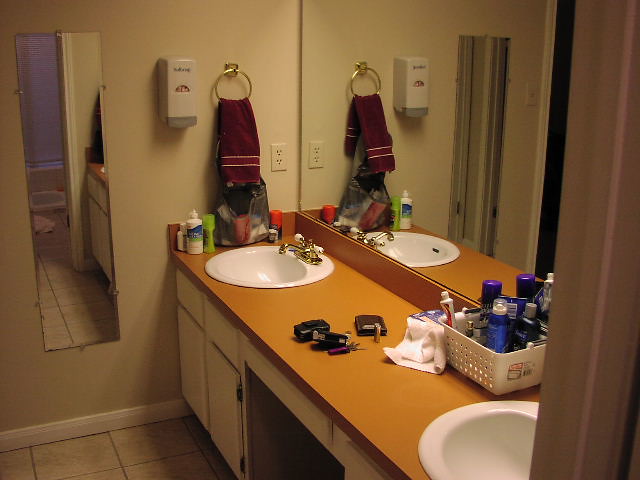A photograph captures the interior of a bathroom featuring a long, orange-colored countertop with two white sinks. The sink furthest from the camera is equipped with a gold-colored faucet and handles, with both hot and cold water handles adorned with white ceramic accents. Mounted on the wall beyond this sink is a gold-colored ring holding a brown hand towel. The other white sink, although partially obscured, likely also features a similar gold fixture. Additionally, a white plastic basket filled with various containers of soap, lotion, antiperspirant, and perfume sits on the countertop, serving as a convenient catch-all for personal care products. Positioned between the two sinks are what appear to be car keys and a wallet, suggesting someone’s pocket items have been temporarily placed there.